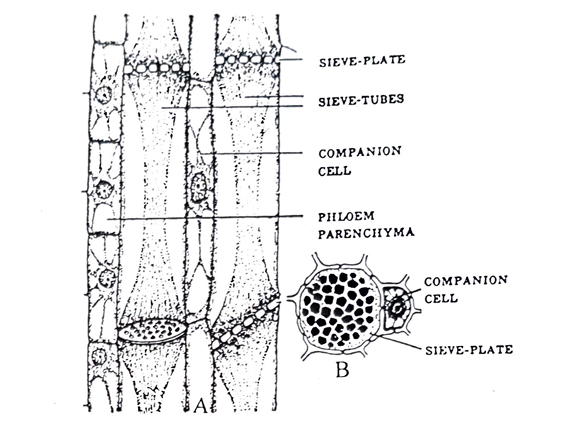This is a black and white, hand-drawn diagram of microscopic cell structures, likely related to plant anatomy though no specific context is provided. The sketch is crude, featuring broken and dotted lines, and is labeled with terms indicative of plant tissue structures. Each labeled part has a horizontal line extending from it. At the top, the label "sieve plate" points to several circular features. Below this, two tubular structures are identified as "sieve tubes," with a shorter horizontal line pointing to one tube. Between the tubes, there's a label for a "companion cell." A line extending from the far left points to an area marked "phloem parenchyma." Additionally, a zoomed-in circular section underneath the main diagram illustrates a closer view labeled "companion cell" and "sieve plate." The overall appearance and style suggest it is educational material typically found in biology textbooks, though specific details about what organism or part of the organism is depicted are not provided.